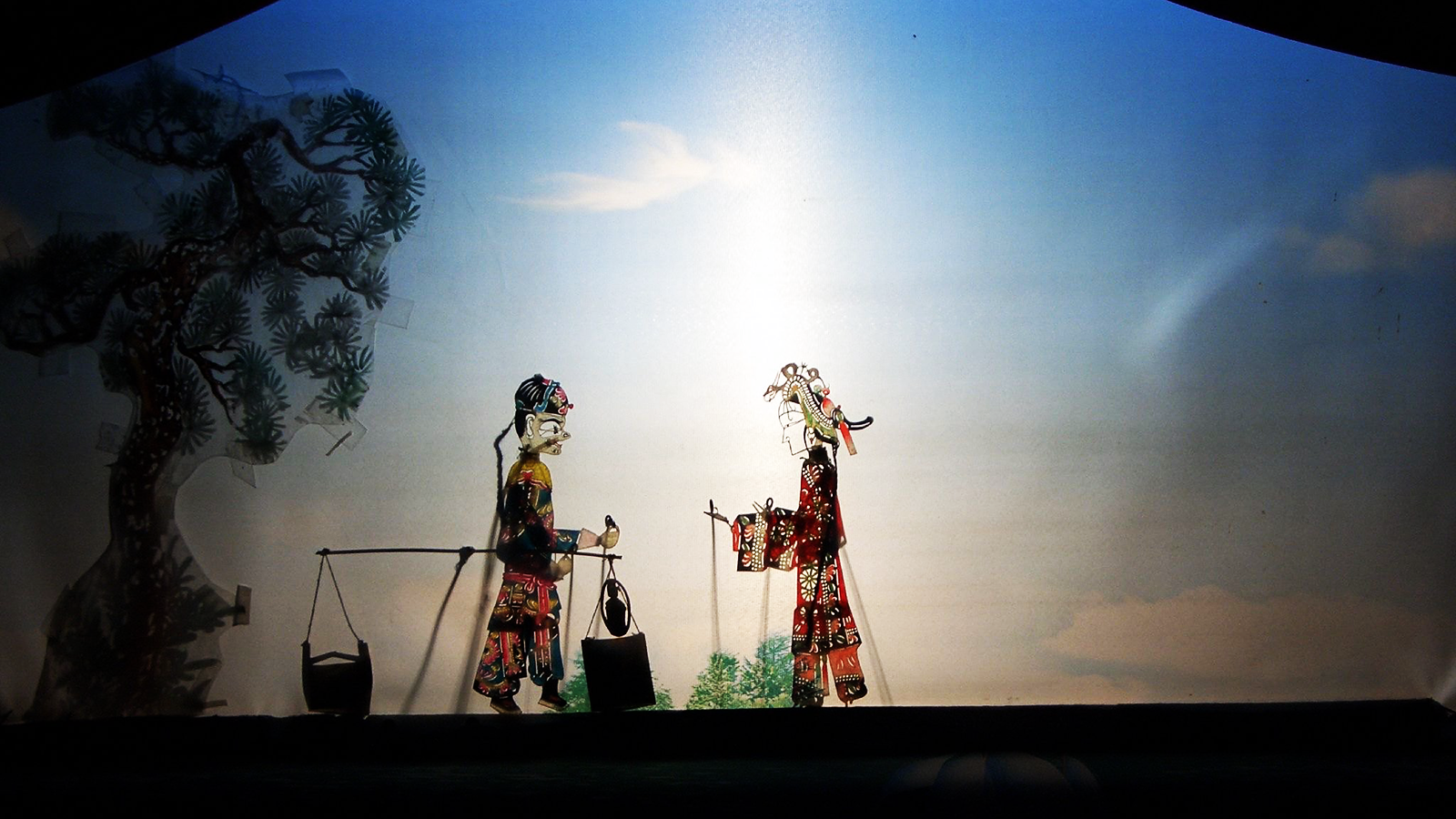The image is a photograph of a large painting set in a dark room, illuminated by a direct light. The painting features a serene outdoor scene with a vibrant blue sky gradually shifting into pale gray clouds. On the left side of the painting is a tree with a dark green, full canopy. The painting primarily depicts two Asian figures dressed in elaborate, multicolored outfits combining patterns of black, red, and white.

The figure on the left, a man with a skin-toned face adorned with prominent white eyes, wears a multicolored hat and traditional oriental clothing. He has a long braid and holds a black satchel with a cord handle in his right hand. Additionally, he carries a stick balanced on his shoulder, from which a black pot is suspended by a rope.

Facing him on the right is a figure that could be a woman, characterized by a peculiar headdress extending down the back, patterned in multicolors of white, black, and red, and a distinct white face. Both figures, in profile, appear to be engaged in a trade or exchange, possibly offering gifts to one another.

Small green plants and scrub bushes populate the background, enhancing the naturalistic setting. The entire painting is set against a black background, reinforcing its presence as an artistic piece mounted on a wall in a dimly lit space.